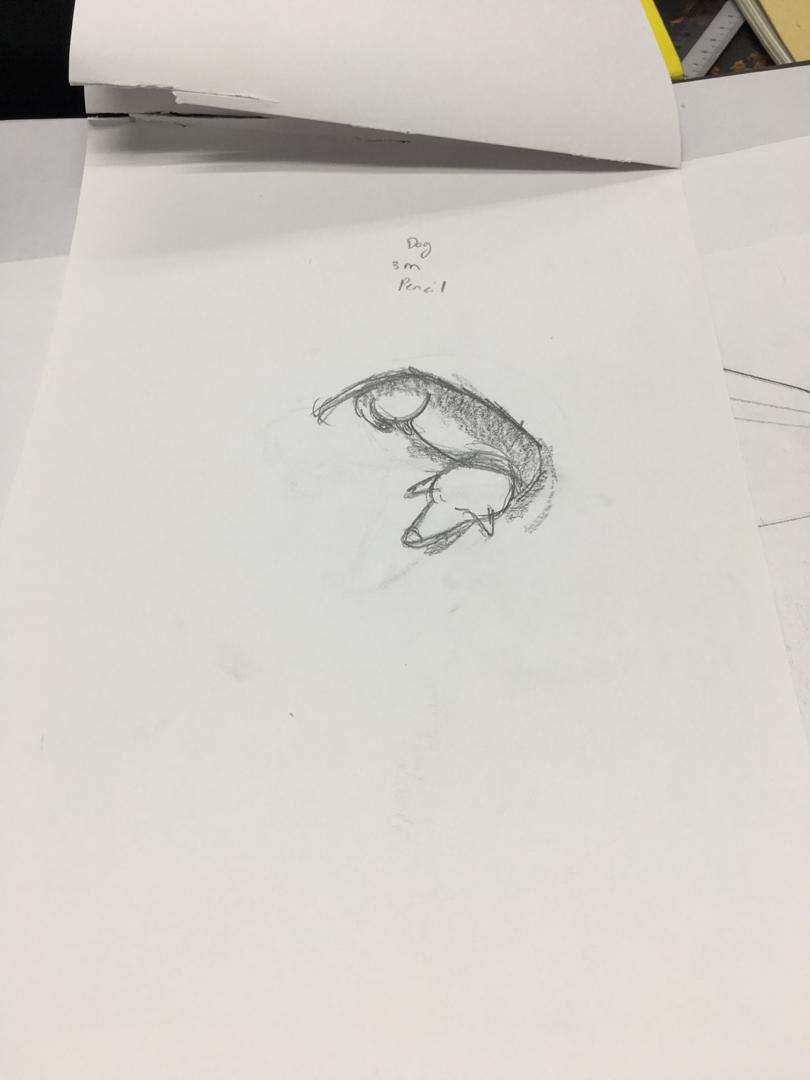The image depicts a vertically oriented photograph that has been rotated 90 degrees to the right, making the new bottom appear on the left-hand side. Dominating the center of the image is a piece of white paper, which is stacked atop multiple other pieces of white paper on a white table. The prominent piece of paper features a detailed pencil sketch. The sketch appears to be of an animal, specifically a dog, rendered with heavy shading and loose sketch lines. The drawing shows the dog in a reclining position, with its eyes closed and head turned to the side. Additionally, the dog is noted to resemble a wiener dog. At the top of this paper, there is some text written in pencil that reads "dog 3M pencil." Various other papers are visible around the edges of the image, and a ruler is situated near the top of the image. Some torn paper is also evident, adding to the overall cluttered but focused scene. The primary focus remains the penciled dog sketch on the topmost piece of paper.